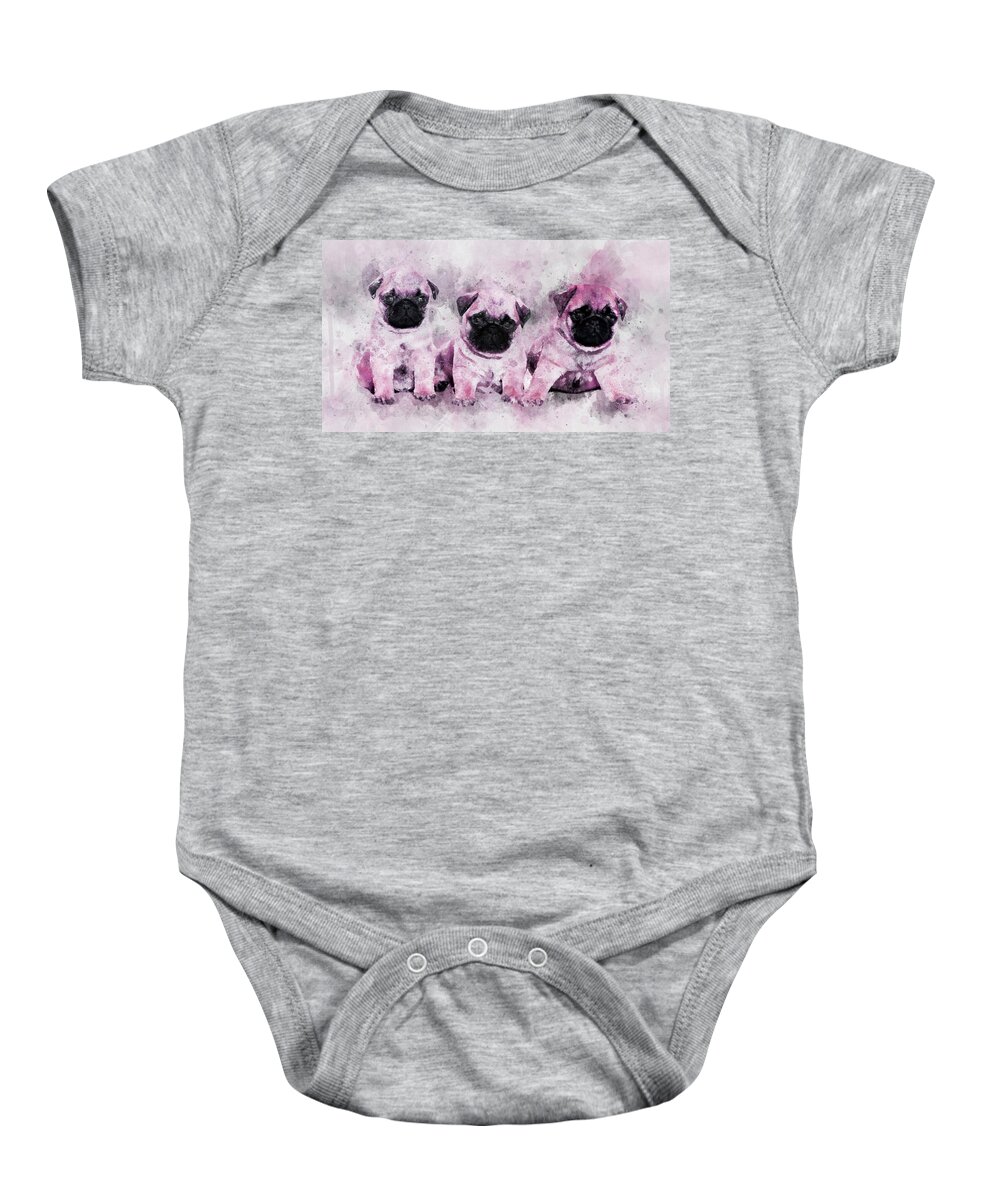This full-color, vertically rectangular photograph showcases a single, staged baby onesie against a plain white background. The gray onesie features short sleeves and a high neckline with a distinctive flap that extends to the front on either side. At the bottom, three small snap buttons secure the crotch area. The central design element is a horizontally rectangular image located just below the neckline, depicting three pug puppies with light brown bodies and black faces, characterized by their smooshed-up noses. These darling puppies sit side by side, facing outward, with dark eyes and hints of black inside their ears. The background of the puppy image includes soft splashes of light pink, adding a gentle, whimsical touch to the well-made, charming onesie.